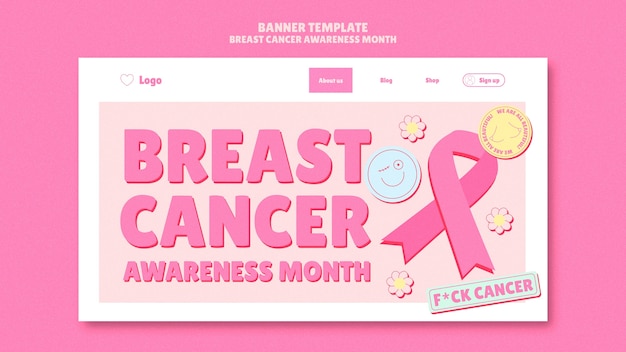The banner is bright pink and promotes Breast Cancer Awareness Month. The main text on the banner reads "Banner Template" in light pink. Below this, in a white square box with shadowing, there's an outlined heart with the word "Logo" prominently displayed in bold pink letters. Adjacent to this box is a smaller pink square with white text that reads "About Us", "Blog", and "Shop". A "Sign Up" button is also featured.

In another section, a light pink square contains bold pink text that says "Breast Cancer Awareness Month". Next to it, a circle with a smiley face represents a breast with one nipple and another sutured out, symbolizing the journey of those affected by breast cancer. Surrounding these elements are various details: a breast cancer awareness pink ribbon, multiple flowers, and a green sign with a pink border that emphatically declares "Fuck Cancer" in bold pink letters. A yellow circle with a pink border and additional text on the periphery adds to the detailed composition of the banner.